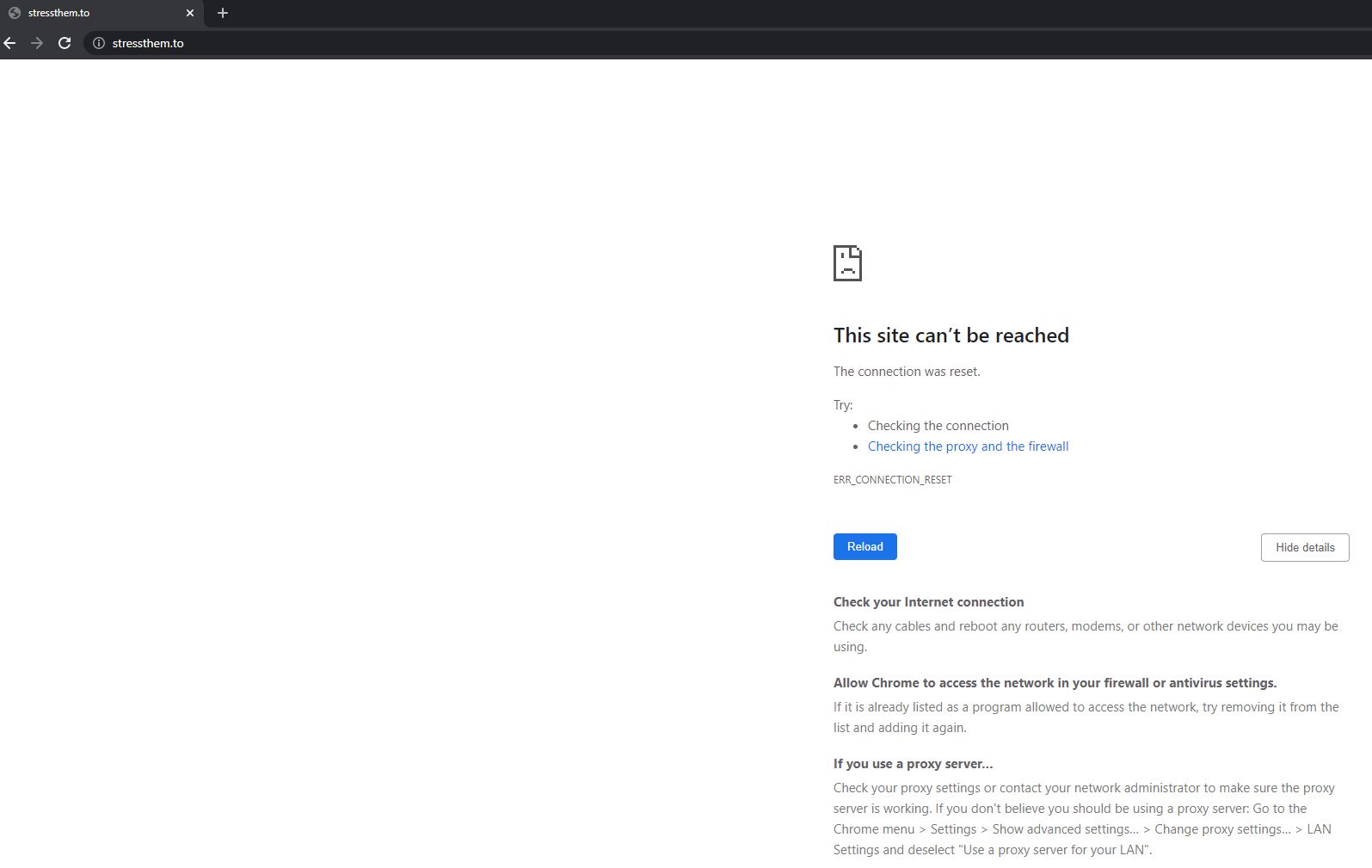A screenshot of a browser window displays the error message "This site can’t be reached." The URL shown is "TrustThem.tl." At the top left, there is a circular refresh button, directional left and right arrows, an "X" button, and a circular icon next to them. In the center of the screen, a document icon with a folded corner and a sad face is visible. The error message indicates that "The connection was reset" with additional troubleshooting steps such as checking the connection, proxy, firewall, and network settings. The error code "ERR_CONNECTION_RESET" is also displayed, with options to "Reload" or "Hide details." The suggested actions include checking the internet connection, cables, and network devices, rebooting routers or modems, allowing Chrome to access the network in the firewall, and adjusting LAN proxy settings in Chrome’s menu.